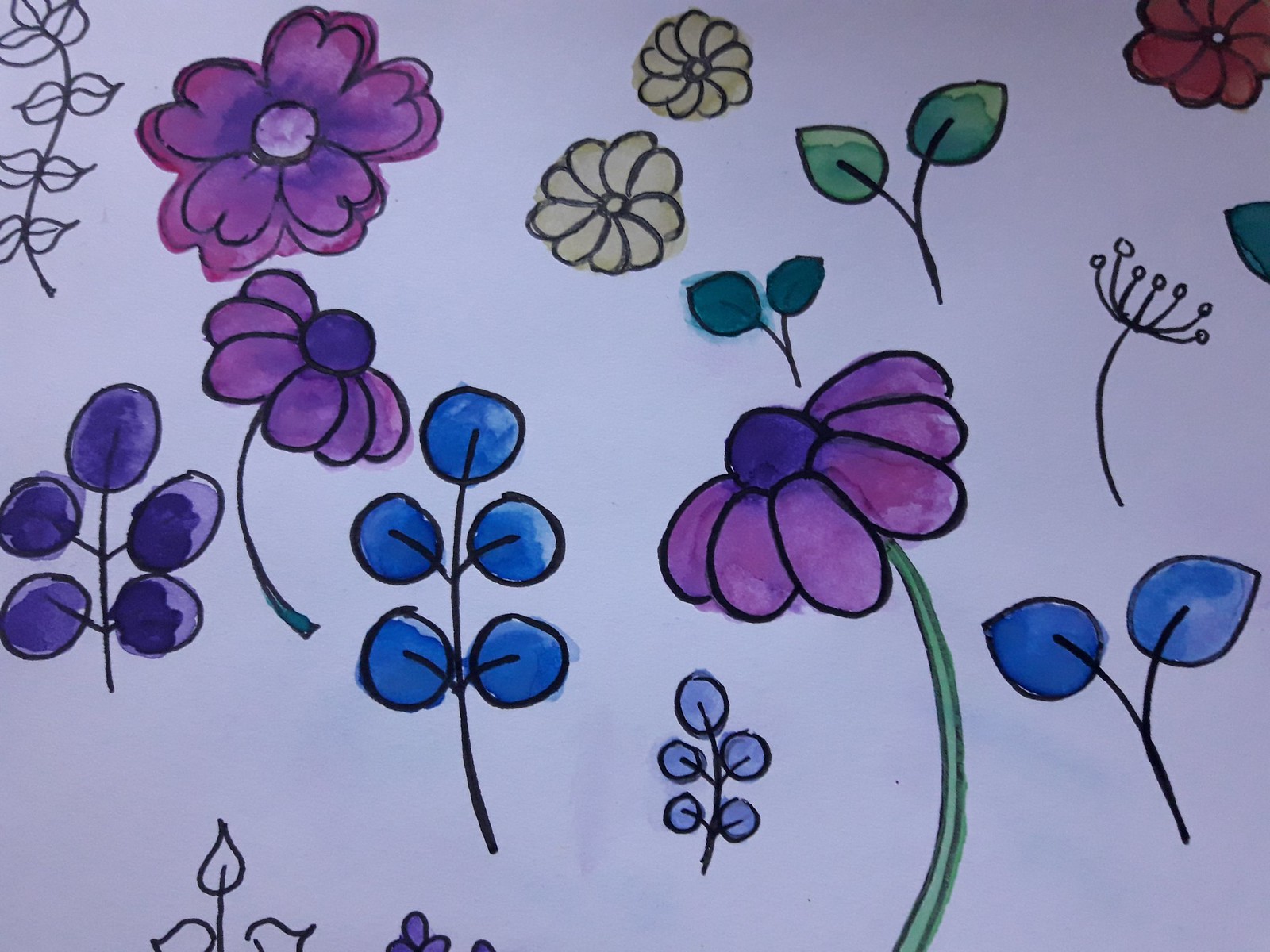This is an artistic rendering of flowers and leaves on a slightly grayish white sheet of paper, likely created using a combination of bold marker outlines and watercolor fills. The arrangement features approximately 10-12 flowers of various sizes and colors, including purple, pink, yellow, and deep red-orange petals. Additionally, numerous leaves, some colored and some left in black ink, complement the flowers. Notably, a small non-colored leaf with alternate leaves appears at the top left, while a purple flower with a blue center and another similarly styled, larger flower are depicted on the right side. Blue plants and purple and blue berries enhance the vibrant scene, with five berries per stem, one on top and four beneath. At the top right, a distinctive red-centered flower with seven petals can be seen. The flowers are illustrated from different perspectives, some viewed from the top and others shown from the side.